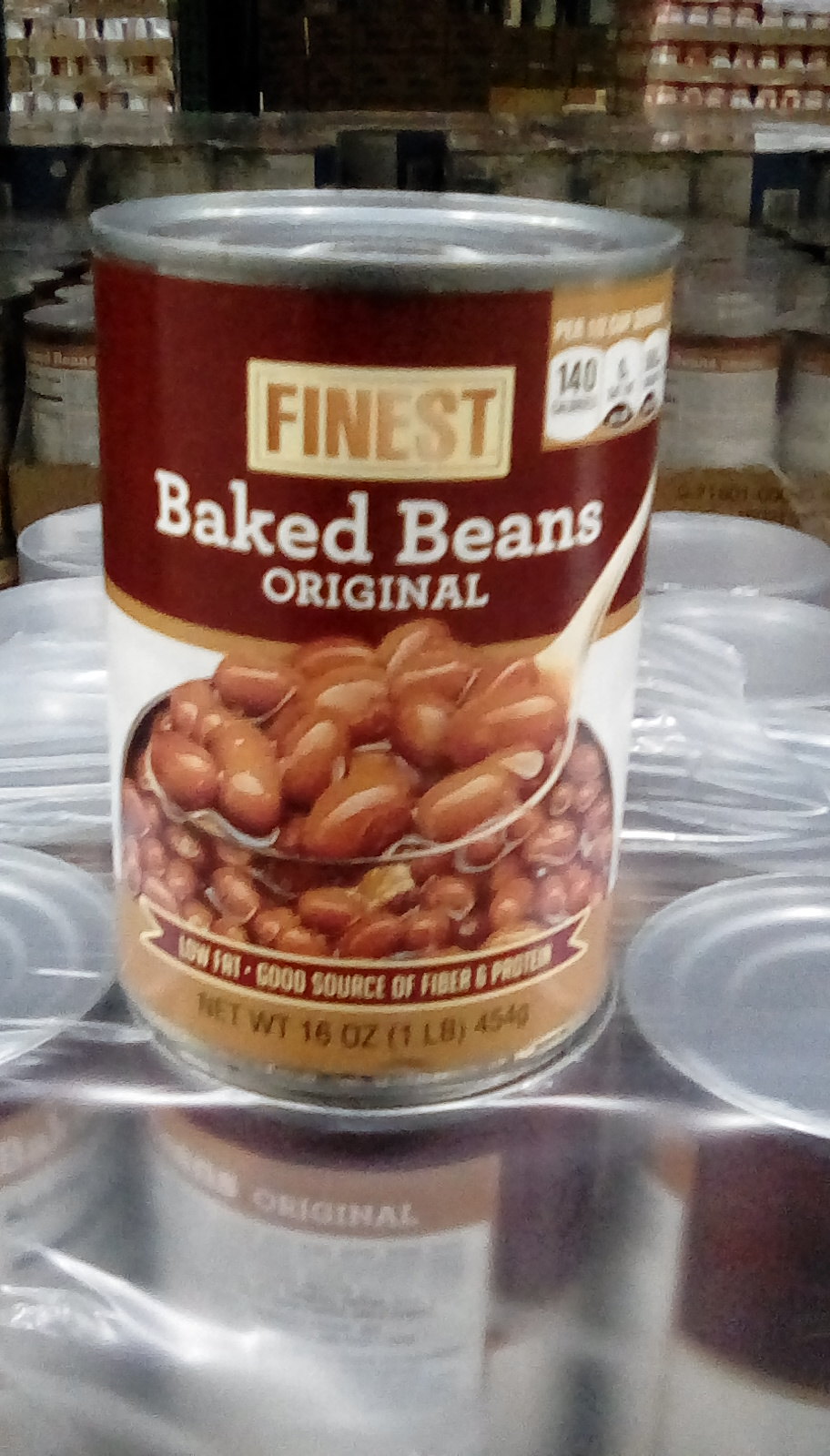This photograph captures a can of baked beans prominently displayed in what appears to be a store or warehouse setting. In the background, pallets can be seen stacked high, alongside flats of canned beans neatly shrink-wrapped in clear plastic. At the center of the image, a single, lone tin can of baked beans stands out. The can features an aluminum body adorned with a distinctive paper label. The label has a burgundy upper section and a white lower section. In the white area, there's a detailed illustration of a bowl of baked beans, accentuated with a spoonful of beans to highlight their texture and appearance. The burgundy top section bears the words "Finest Baked Beans, Original." The composition and lighting emphasize both the product and its industrial surroundings, creating a vivid and detailed depiction of the scene.